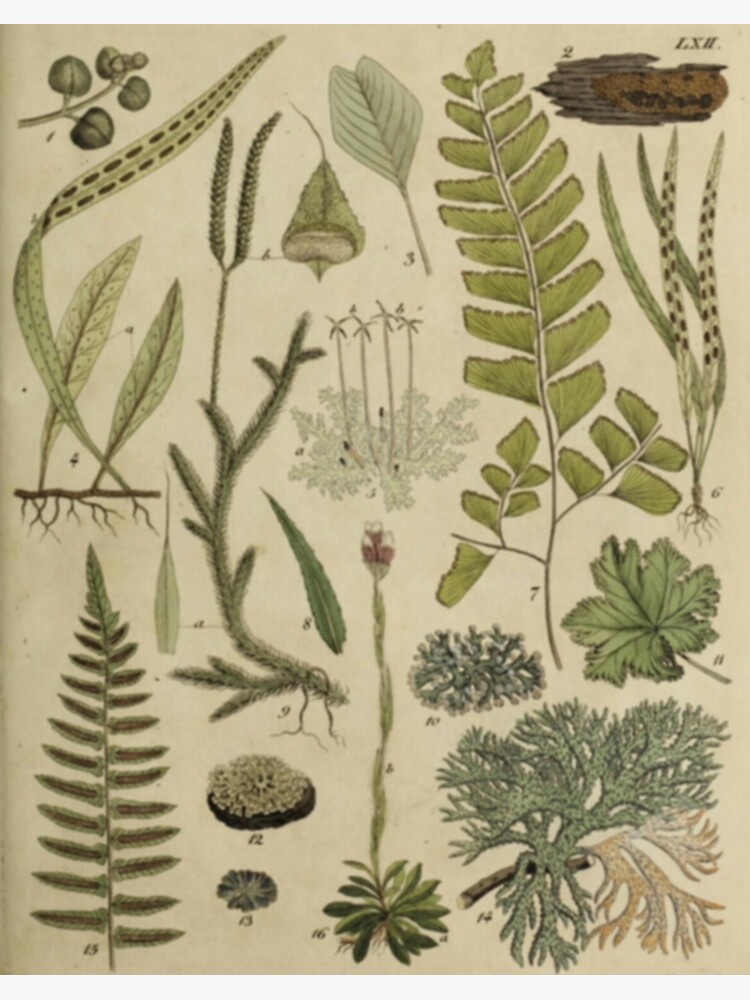This image depicts a detailed botanical drawing of various types of flora, primarily characterized by shades of green and brown against a cream-colored background. The illustration showcases a variety of plants, including what appear to be aquatic species or those commonly found in wet environments. Each plant is meticulously drawn, displaying not only the leaves but also roots, with several specimens appearing similar to ferns, corals, or grasses.

Numbered annotations accompany each plant, suggesting the presence of a legend likely on a separate page. In the top left corner, there are small spade-shaped leaves and what appear to be tiny acorns or buds. Adjacent to it, a section labeled "two" displays a piece of bark. As the eye moves downward, a slender leaf with visible roots is illustrated, followed by a more fir-like leaf and various rounded, spade-shaped, or elongated leaves.

One prominent plant in the middle of the image has roots and polka-dotted leaves with dark hash marks along the spine, hinting at its grass-like nature. Another specimen on the right side features a fuzzy, tendril-covered plant, also showcasing its root system. At the bottom right, there is a partly decaying, lettuce-like leaf.

The detailed illustration includes a long branch with numerous offshoots on both sides, resembling a complex network of leaves. Additionally, a leaf reminiscent of a jagged-edged maple appears, along with a bushy plant exhibiting both green and orange hues, indicating a mix of vitality and decay. Among other identified flora are lily pads, a fern stalk, a pink flower with white tips atop a long stalk, and a mushroom-like specimen with white filaments and dark base.

Overall, the botanical drawing is a comprehensive and intricate depiction of diverse plant types, providing a visually rich exploration of their forms and structures.